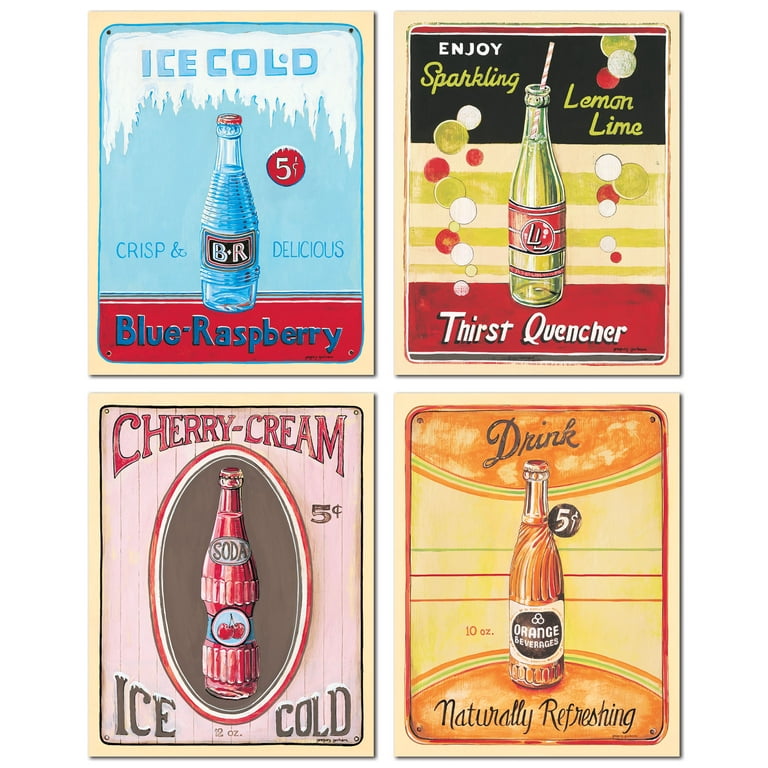This image features a nostalgic collection of four vintage soda advertisements arranged in a 2x2 pattern, resembling old tin signs or wall art. Each rectangular sign shares a beige border.

- **Top Left**: "Ice Cold Blue Raspberry" showcased in an ice cube-themed design. A blue glass bottle, with the label marked "BR" in blue, advertises the flavor for 5 cents.
- **Top Right**: "Sparkling Lemon Lime" branded as a thirst quencher, features a green bottle with white and red accents in a greenish backdrop. The label, denoted "LL," includes a red rectangle at the bottom.
- **Bottom Left**: "Cherry Cream Ice Cold Soda," also priced at 5 cents, is a bright red bottle adorned with cherries. The label highlights "ice cold" below the image.
- **Bottom Right**: An orange beverage titled "Drink Naturally Refreshing." This orange glass bottle is set in an orange-themed design, emphasizing its refreshing quality.

The collage evokes a mid-20th century aesthetic, reminiscent of the 1950s and 1960s soda vending machine advertisements.